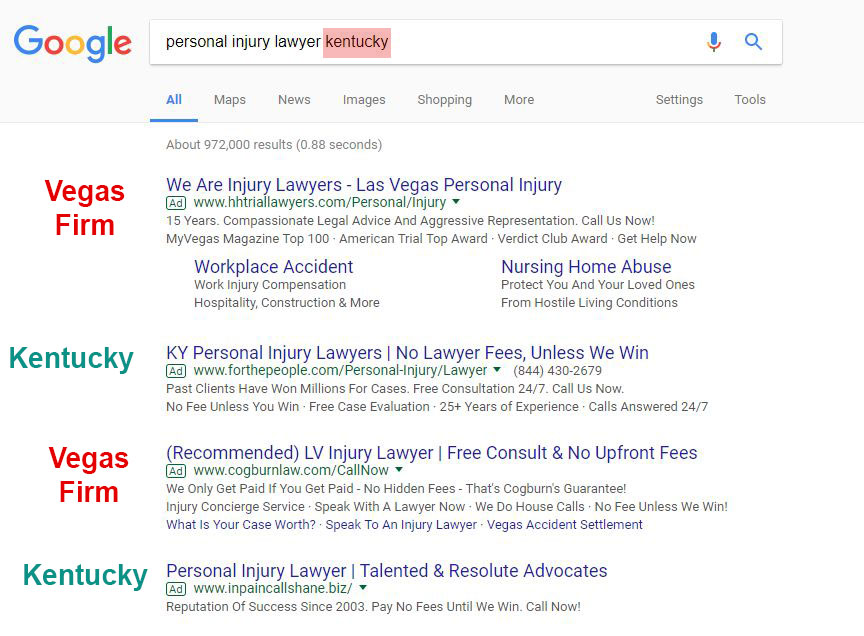In this image, the Google search results for the query "personal injury lawyer Kentucky" are displayed. Positioned to the right of the search bar is a microphone or speech icon, alongside a search icon depicted as a magnifying glass. On the left side of the search bar, the multi-colored Google logo is prominently featured in blue, red, yellow, and green. The search has yielded approximately 972,000 results in just 0.88 seconds. 

Several links are visible, including a few that are not directly related to Kentucky, such as "We Are Injury Lawyers," which highlights their services in Las Vegas, noting 15 years of compassionate legal advice and aggressive representation, with awards like "My Vegas Magazine Top 100," and "American Trial Top Award." Phrases like "Call us now" and "Get help now" are also mentioned.

Text on the left sidebar reads "Vegas Fame" and "Kentucky." The page shows four primary search results:

1. "Personal Injury Lawyer - Silenced and Resolute Advocates."
2. "KY Personal Injury Lawyers - No Lawyer Fees Unless We Win."
3. "Recommended LV Injury Lawyer - Free Consults and No Upfront Fees."

This detailed description emphasizes the search interface and the nature of the search results displayed on the page.